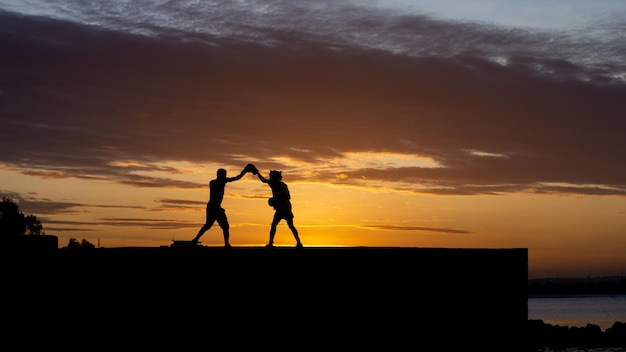Beneath a dramatic sunset, with the sky painted in hues of orange and gray, stands a silhouetted scene captured in this horizontal photograph. Dominating the foreground is a flat, black platform, possibly a rooftop or a wall, with a sharp drop-off. Atop this platform, two boxers in black silhouette, their arms extended upwards, touch gloves in a gesture that suggests either sparring or camaraderie. Their dark forms are striking against the bright, backlit sky. Stretching across the middle of the distant horizon, the sun's glow illuminates the scene without appearing directly in the frame. Dark, elongated clouds hang in the sky, contributing to the moody atmosphere. To the left, the faint outlines of trees are visible, while the bottom right corner hints at the presence of a body of water, adding depth to the tranquil yet intense setting.